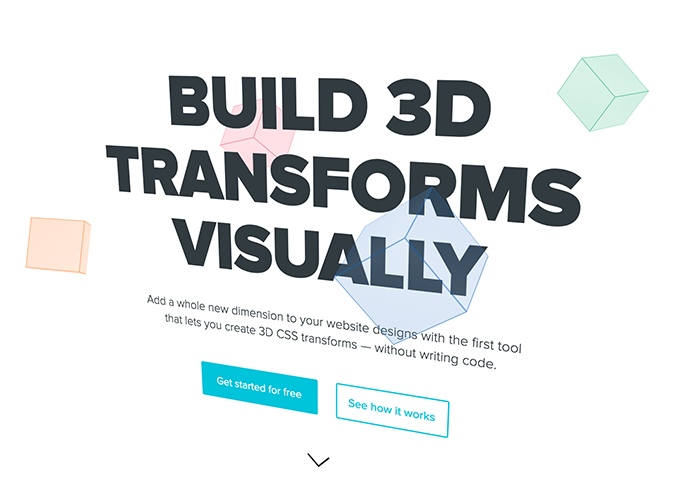The image is a piece of vector art presented at an oblique angle, giving it a dynamic perspective where the right side appears closer than the left. 

Centered in the artwork is bold, all-caps text that reads "BUILD 3D TRANSFORMS VISUALLY." Below this headline, in smaller text, it states: "Add a whole new dimension to your website designs with the first tool that lets you create 3D CSS transforms—without writing code." 

On the left side of this text block are two buttons. The first button is a solid teal color with white text saying "Get Started For Free." The second button has a teal outline and a white background with teal text that reads "See How It Works." A dark grey arrow points downward, drawing attention to these interactive elements.

In the background, four differently colored cubes illustrate the 3D transform capability. From left to right:
  
1. An orange cube with its front face prominently visible.
2. A red cube positioned at an equal distance to the right of the orange cube, viewed from the side.
3. A blue cube also shown from the side, placed rightward of the red cube.
4. A green cube, slightly closer than the red and orange ones, floating on the far right.

Together, these elements visually convey the tool's ability to create and manipulate 3D effects without the need for coding.